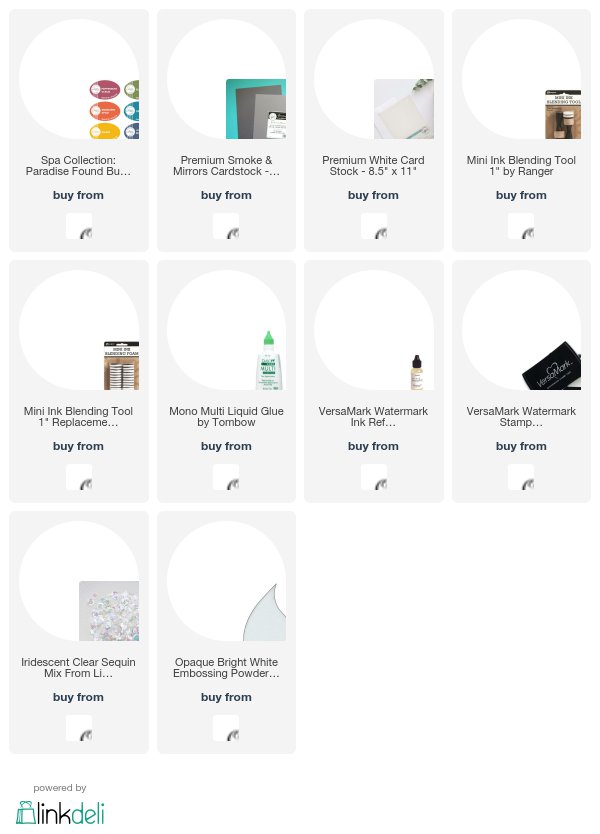The image depicts a section of a website, presumably belonging to a company named Link Deli. The logo, displayed at the top, consists of "Link" in black and "Deli" in green, preceded by a green shopping bag icon. The layout features several individual gray boxes, each containing a product image within a white circle. Unfortunately, the product images are misaligned, being positioned towards the lower right side of their respective circles.

In the top row, the first product's label is partially cut off. It reads "Spa Collection, Paradise found" with the visible portion ending abruptly. Following this, there is an item described as "premium smoke and mirrors card stock." Additional products in this row include "premium white card stock" and a "mini ink blending tool."

The second row continues with similar issues in image alignment, showcasing items such as a "mini ink blending tool" one-inch replacement, "mono multi-liquid glue," "VersaMark watermark ink," "VersaMark watermark stamp," "Indescent clear sequins," and "opaque bright white embossing powder."

The overall presentation of the products is poorly executed, with cut-off labels and misaligned images detracting from the viewing experience. The website appears to need substantial improvement in its product display and layout management.